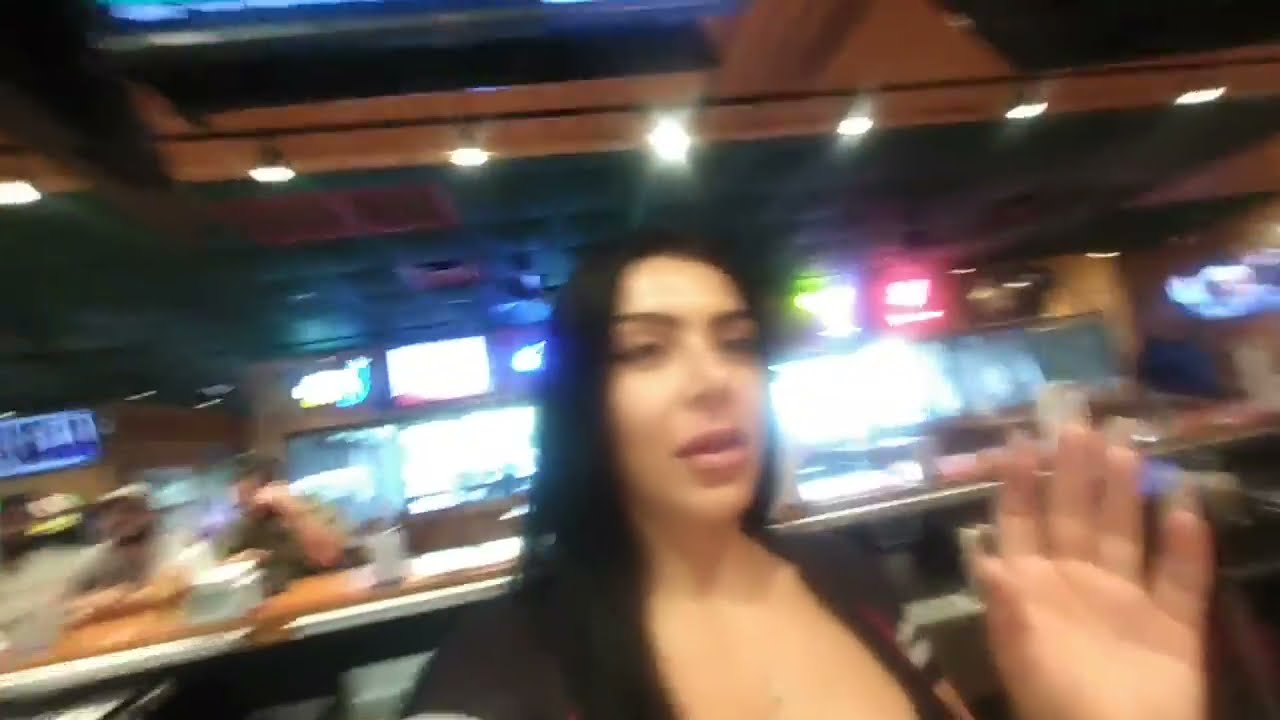The photograph captures a woman indoors, likely in a bar or restaurant setting. Due to movement, the image is notably blurry, distorting definitive shapes and details. The woman, who has a medium to light tan skin tone, is positioned centrally and slightly turned to the right, with her left hand raised as if to avoid having her picture taken. She has long, straight black hair that extends past her shoulders, dark eyebrows, eyes, full lips, and a straight nose. Dressed in a low-cut black top, she appears in motion, heightening the blurriness. 

The backdrop consists of a bar counter with a few indistinct figures seated, partially illuminated by bright lights that contribute to the overall whitewashed appearance of the background. Above the bar area, the ceiling displays spotlights and materials that seem wooden. Additional lights cast colorful hues, including pink, in the surroundings. There are also several television screens visible in the blurred background, enhancing the lively bar atmosphere. Despite the lack of text or clear focus, the scene is vibrant and dynamic, suggesting a bustling social environment.